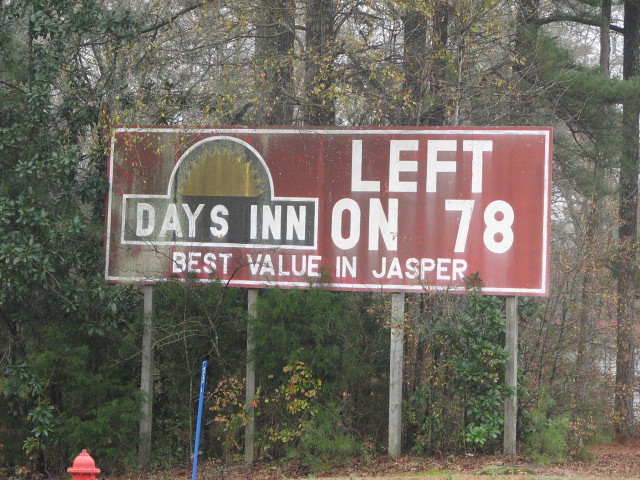A roadside billboard stands amidst towering trees, their greenery interspersed with autumnal hues of yellow and orange, indicating the fall season. Fallen orange leaves carpet the ground. The sign, supported by four wooden beams, features a red background. On the left side, the Days Inn logo is prominently displayed. Beside the logo, white text directs travelers to turn "left on 78," and below, it boasts "Best Value in Jasper." In the bottom left corner of the photograph, a red fire hydrant and a blue pole are visible, adding to the scene's detail.